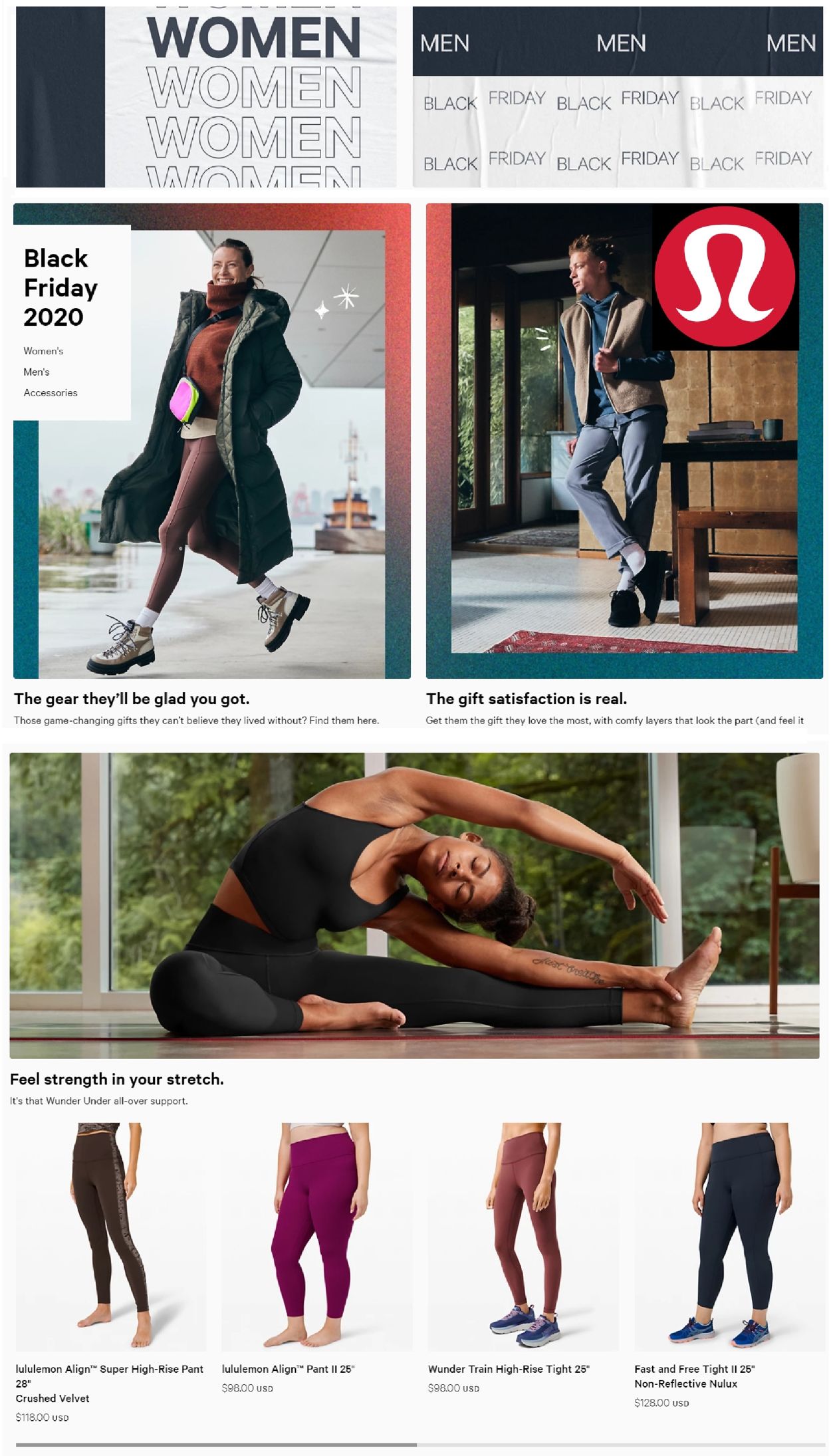This vertical web image prominently features a Black Friday promotional banner from Lululemon. At the top, there is a light black and grayish vertical stripe running downwards, followed by a white box repeatedly displaying the word "women" in alternating blackish-gray and white fonts. Below this, a horizontal light black box features the word "men" in white, repeated several times. The area beneath this has "Black Friday" text repeatedly displayed against a light gray background, emphasizing the 2020 Black Friday event.

Further down, the image showcases a collage of rectangular photos, some aligned vertically and others horizontally, depicting various models dressed in Lululemon clothing. The iconic red circle with the white Lululemon logo is visible in the upper right corner of one of these model photos. Accompanying captions include motivational phrases like "The gear they'll be glad you got," "The gift satisfaction is real," and "Feel strength in your stretch."

In the lower section of the image, there is a feature of four distinct pairs of yoga pants, each with its title and price listed below. Additionally, a model performing yoga poses prominently highlights the functionality and style of the workout attire.